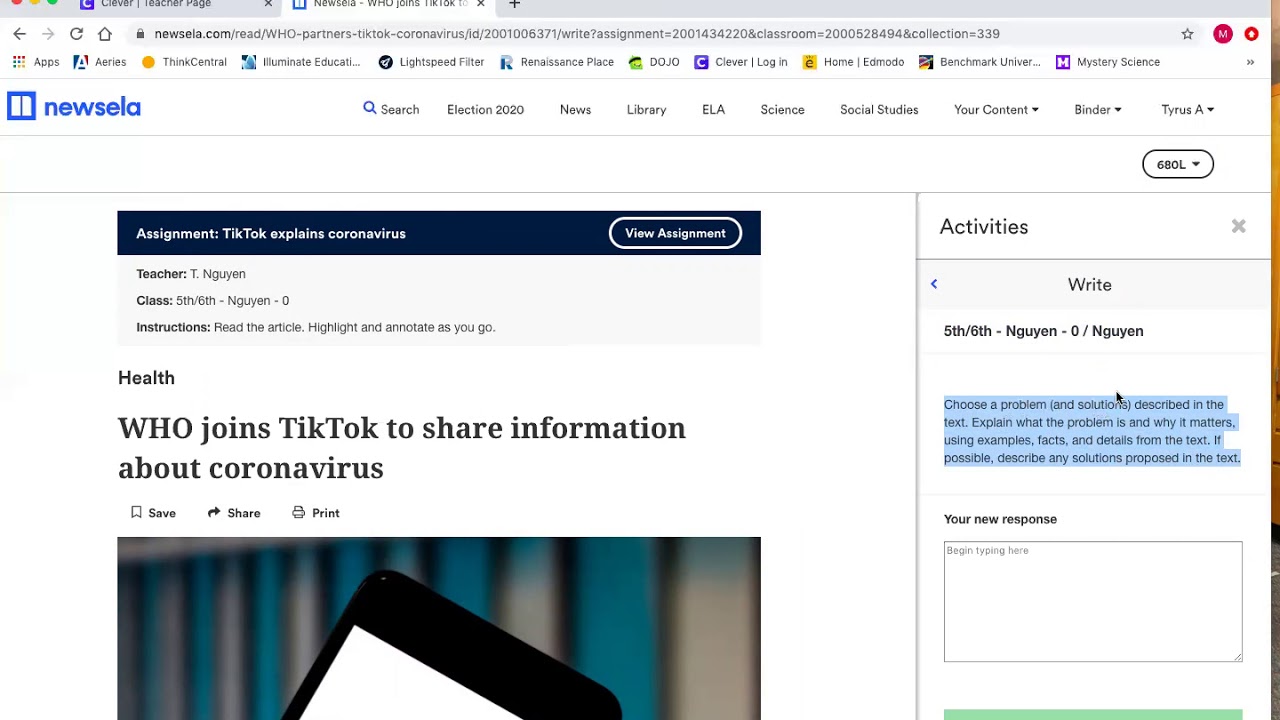This image showcases the user interface of a website, seemingly accessed on an Apple product. At the top of the page, partially cut-off circles indicate the typical red, yellow, and green window control buttons of macOS. To the right of these buttons, there's a partially visible blue box with what appears to be a cut-off letter "C". The browser tab itself is also slightly obscured but reveals a plus sign on the right.

Directly below, on the left side, there is a highlighted left-pointing arrow. Next to it, a right-pointing arrow appears grayed out, followed by a refresh symbol and a house icon. The search bar, prominently displaying the web address, is positioned centrally, flanked by various favorite apps and bookmarked pages on the favorites bar.

The primary content section features "Newsela" with its blue book icon, prominently displayed on the left. Adjacent to it is a main article with navigation options: "search," "election," "2020," "news," "library," "ELA," "science," "social studies," "your content" with a drop-down arrow, "finder" with a drop-down arrow, and "Tyrus A" with a drop-down arrow.

Beneath this header, the article titled "Who joins TikTok to share information about coronavirus" is aligned towards the left with a partially obscured phone image beneath. Above this title is an oval-shaped button labeled "View Assignments." To the right, the section is labeled "Activities," and centrally aligned below it, the word "Write" is displayed. Further down, the text "5th, 6th, Nugent" is followed by a highlighted paragraph section. A prompt for "your new response" is situated above a blank text box, inviting user input.